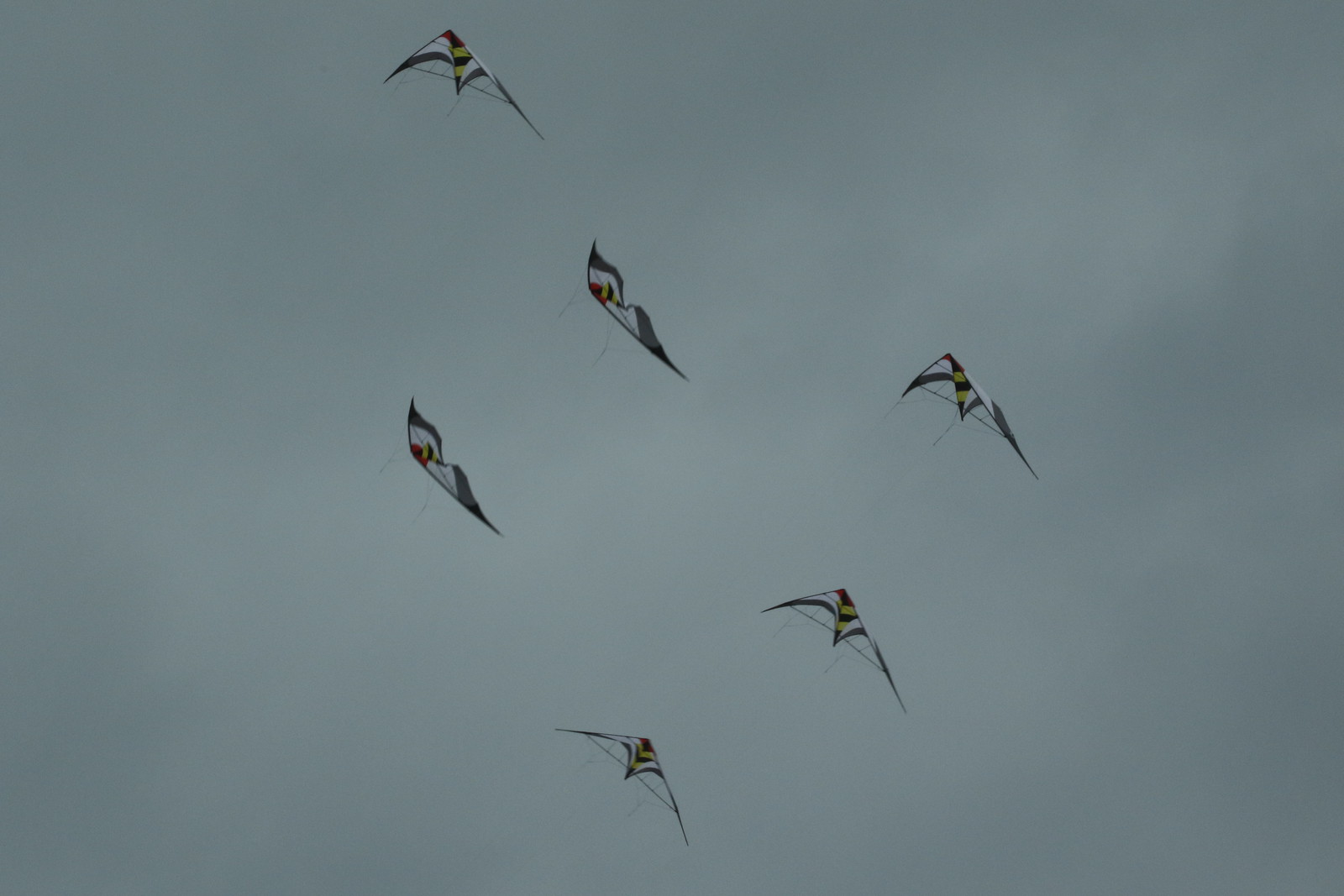This photograph, wider than it is tall, captures a scene of six triangular kites soaring in a gray, overcast sky without a hint of blue or sunlight. The kites are arranged in three tiers across the middle section of the image. At the top left, there is a single kite with red at its nose, followed by white and green stripes. Below it, two kites positioned side-by-side have similar triangular shapes and colors, featuring red tips and blue wing edges. These kites are headed towards the left. The bottom tier consists of three kites aligned in a row, flying upwards to the right. These kites showcase stripes of yellow, black, red, and white. The background's gray hues blend with some white shading, suggesting clouds, and the overall scene is free of people or the ground, focusing solely on the kites suspended in the sky.